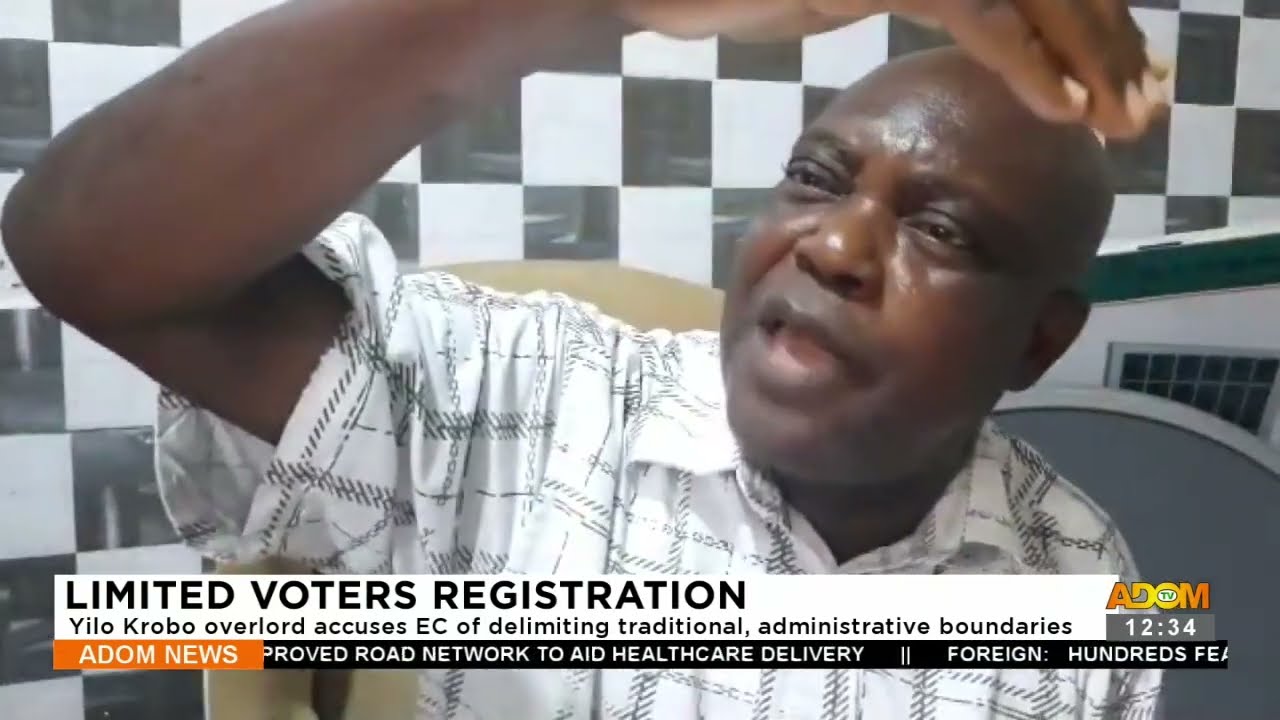The image is a detailed screencap from a television broadcast showing an animated African-American man in mid-speech. He is captured from the chest up, emphasizing his expressive motion with his right arm raised above his head, his hand partially out of the frame. His face is turned slightly to the side, mouth open as if speaking passionately. He wears a white polo shirt adorned with distinctive black, ragged and jagged cross-cross patterns. The backdrop features a distinctive black-and-white checkered wall on one side and a plain white wall with a vent or register on the other. At the bottom of the screencap, a banner in black text on a white background reads, "Limited Voters Registration. Yilo Krobo Overlord accuses EC of delimiting traditional administrative boundaries." Beneath this, there is a red rectangular box with the brand "ADOM News" in white text, and a black rectangle stating “Approved road network to aid healthcare delivery, foreign hundreds.” The ADOM logo appears in orange, along with a timestamp in white text on a gray bar showing "12:34."